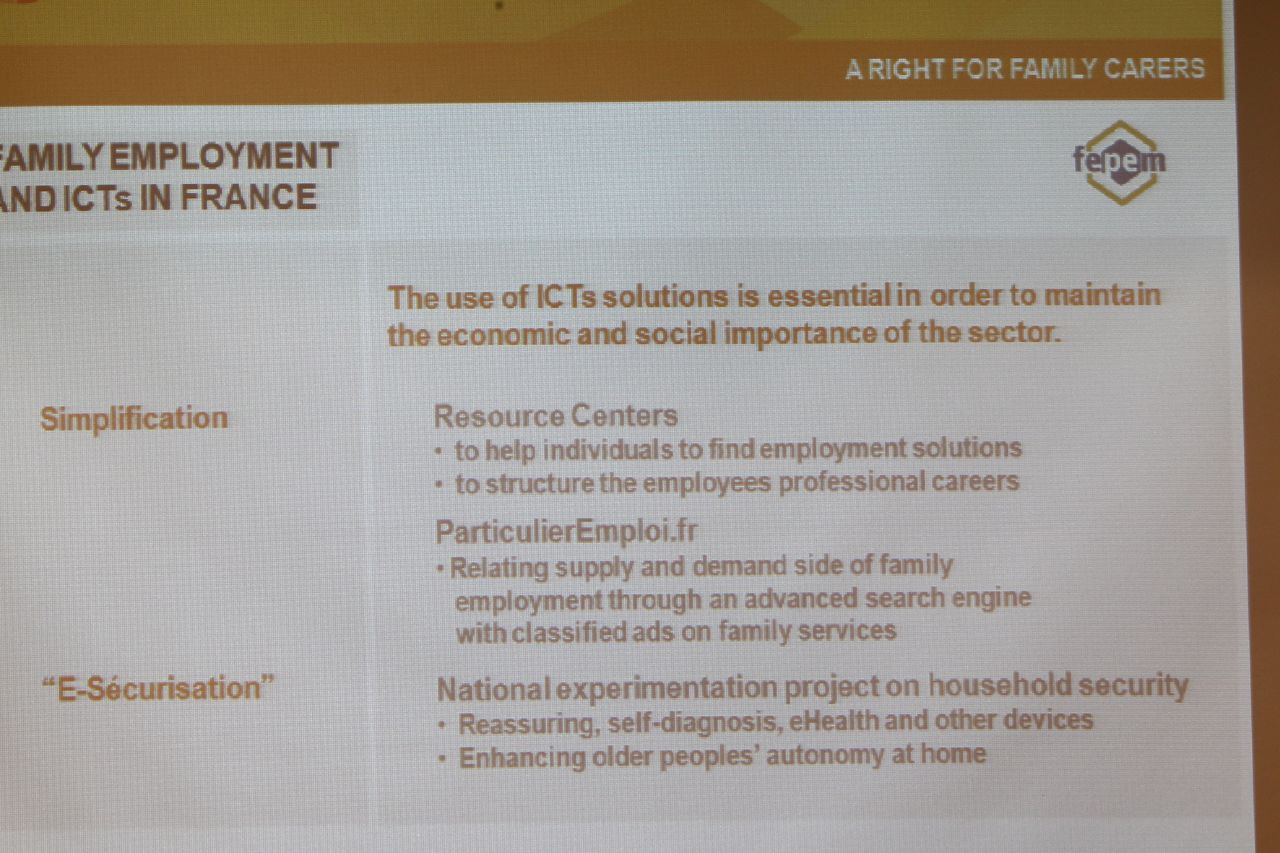The image depicts an online screen display, possibly from a computer monitor or kiosk. The background is predominantly white with an orange or brown line running horizontally at the top. On the right side of the line, in white text, is the phrase "A right for family carers," followed by the acronym "FEPEM," which stands for Family Employment and ICTs in France, depicted within a hexagon-shaped logo in gray and white letters.

On the left side of the screen, the text reads "Family Employment and ICTs in France," with the terms "Simplification" and "E-Securisation" appearing just below, likely written in French. It emphasizes that the use of ICT solutions is crucial for maintaining the economic and social significance of this sector.

Beneath this, in gray letters, it mentions "Resource Centres to help individuals find employment solutions to structure the employees' professional careers," highlighting the role of the website ParticulierEmploy.fr. This site connects the supply and demand sides of family employment via an advanced search engine featuring classified ads on family services.

Towards the bottom, the image details a "National Experimentation Project on Household Security," which includes reassuring self-diagnosis, e-health initiatives, and other devices aimed at enhancing older people's autonomy at home.